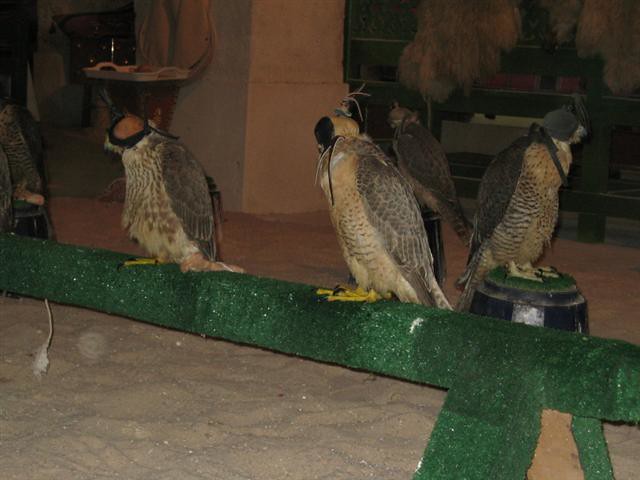The photograph is a horizontally oriented image, resembling a realistic shot. It is predominantly dark and poorly lit, making it somewhat difficult to distinguish fine details. The background features what appears to be a building structure, possibly with concrete walls suggesting an outdoor setting. The ground below seems to be covered with sand, which contributes to the impression of an outdoor environment, perhaps a falcon training area.

Dominating the foreground, a thick green horizontal wooden bar, supported on one end by green legs, stretches from the left side of the image downward to the bottom right. Perched on this bar are four large birds resembling hawks. These birds have gray wings folded by their sides, white and beige chests with speckled dark brown lines. Each bird's head is hooded in a black covering that obscures their faces. Their feet are yellow, adorned with black claws.

Apart from the two birds on the horizontal bar, two more birds are visible, each perched on separate small circular black platforms topped with faux grass. In the left part of the background, some fabric-like items are hanging, possibly a tray, while on the dark right side, there seems to be wooden furniture or some structure adding to the complexity of the scene.